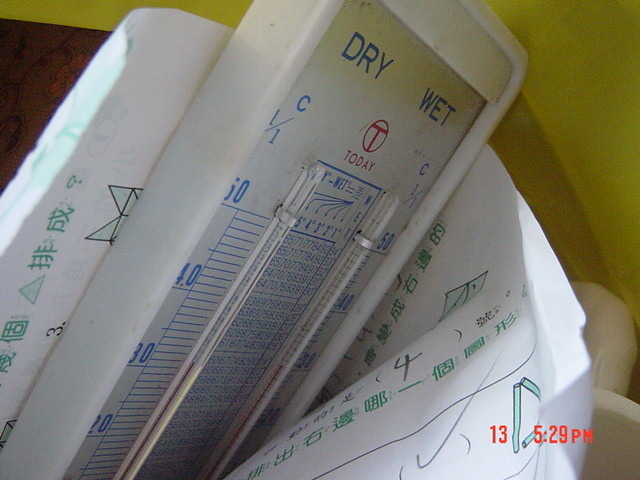The image showcases a highly magnified view of an object featuring numeric data and various charts. In the bottom right corner, the numbers "13" and "5:29 PM" appear in orange text. Directly above is a white piece of paper partially obscured by a gray shadow, predominantly on the left side. Green symbols line the outer edge of the image, with the number "4" displayed in black text above them. Another set of green text is present within the interior of the paper. 

On the right side, a tan cushion is visible, set against a lime green wall background that extends to the top right corner. To the left of the green text, a rectangular-shaped tool is marked with blue numbers along the left side, descending from 50 to 40, 30, and then 20. Adjacent to these numbers are horizontal blue lines. The center of the image contains a series of extremely small numbers. On the right, the same sequence of blue numbers, descending from 50 to 20, is repeated. A central symbol depicting a “T” is accompanied by the word "today." Two words are positioned at the top corners; "dry" on the top left, and "wet" on the top right, with a blue "C" and a "1/1" situated below these words.

The white paper extends around the object, and the background transitions from the lime green wall to a brown section below.